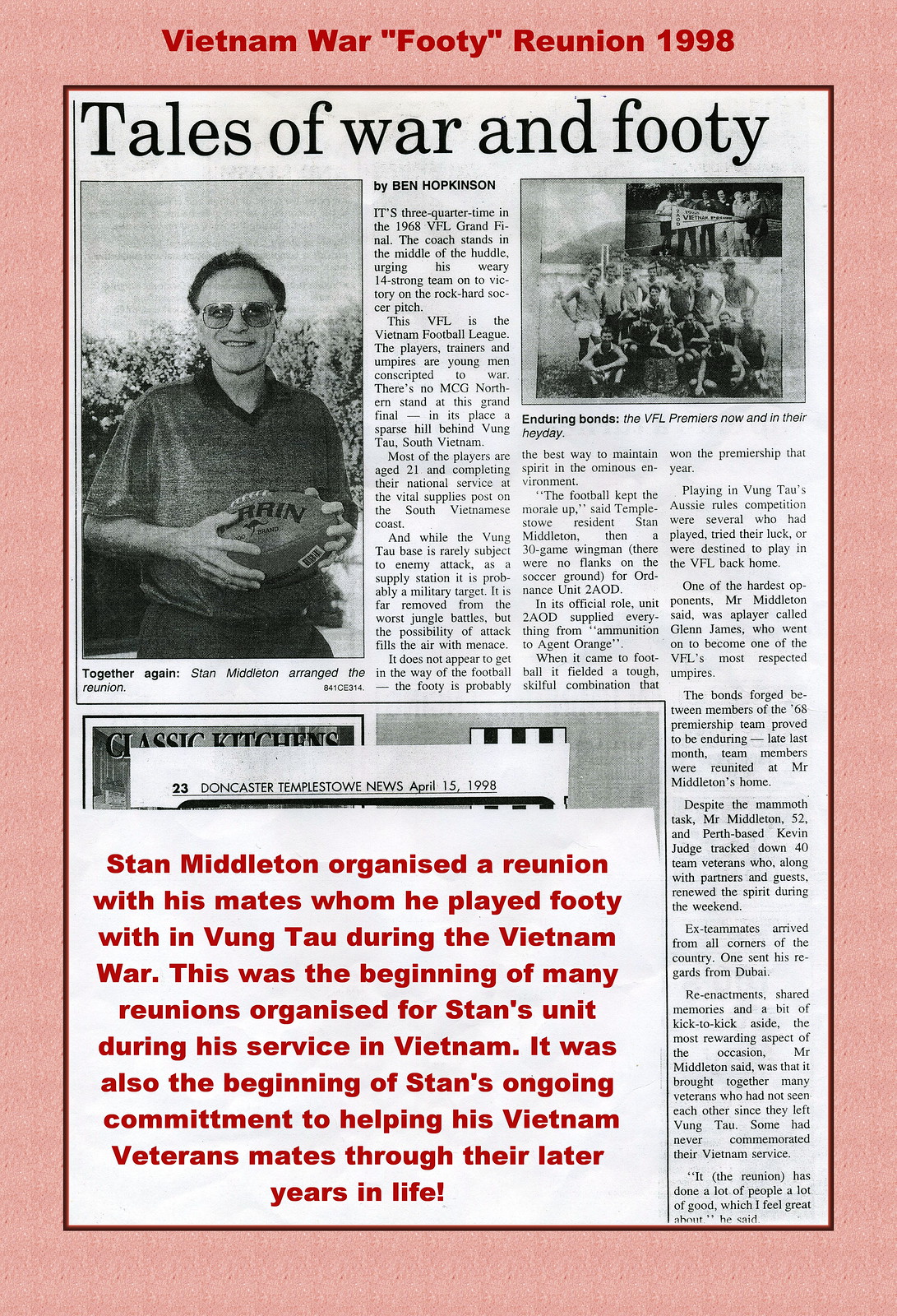The image depicts a photocopied newspaper page set against a pink background, framed by a red border that reads, "Vietnam War Footy Reunion 1998." The article, titled "Tales of War and Footy" by Ben Hopkinson, is presented on a white background with black text. Prominently featured on the left side is a black-and-white photo of Stan Middleton, wearing aviator glasses and a collared short-sleeved shirt tucked into his pants, holding a football. Below his photo, the caption states, "Together again, Stan Middleton arranged the reunion." In the upper right corner, there's another black-and-white photo showing a football team with the caption, "Enduring Bonds, the VFL premieres now and in their heyday." Overlaying the article’s text is a white square with red text that reads, "Stan Middleton organized a reunion with his mates whom he played footy with in Vung Tau during the Vietnam War. This was the beginning of many reunions organized for Stan's unit during his service in Vietnam. It was also the beginning of Stan's ongoing commitment to helping his Vietnam veteran mates through their later years in life."